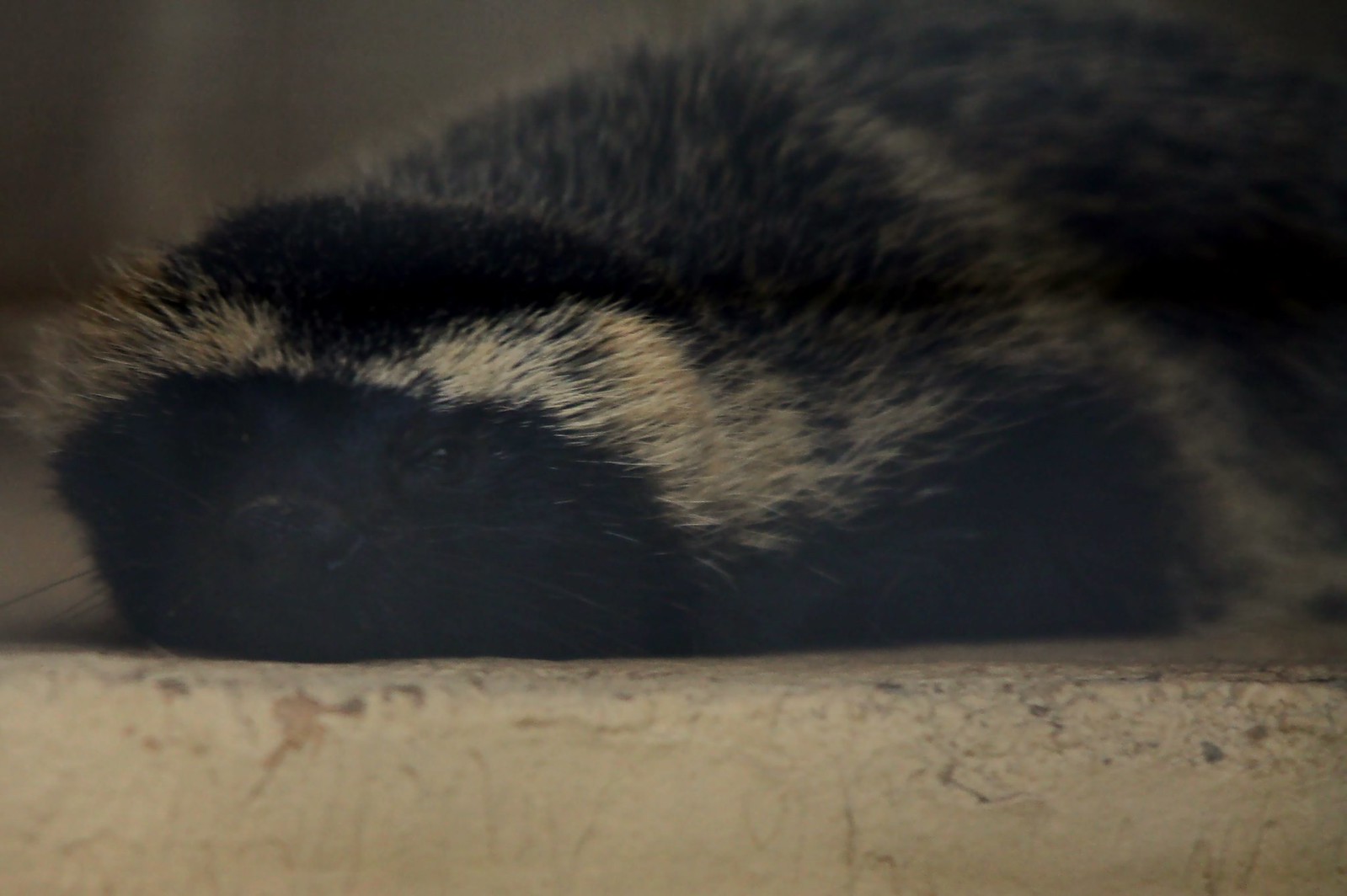The image depicts a close-up of an animal resembling a skunk, lying on a cracked, cream-colored floor with visible pockmarks where the paint has worn away. The animal's body is predominantly black with a white stripe running over its eyes and extending possibly to its back leg, although its body appears to have a salt-and-pepper mix of colors. Its face, with dark eyes and a very black nose, is the focal point of the photo, staring directly into the camera, though the details are somewhat blurred and out of focus. Whiskers are visible, adding to the indistinct yet palpable features of fatigue or contentment. The background appears grayish and slightly out-of-focus, emphasizing the wear and tear of the surface it rests on.